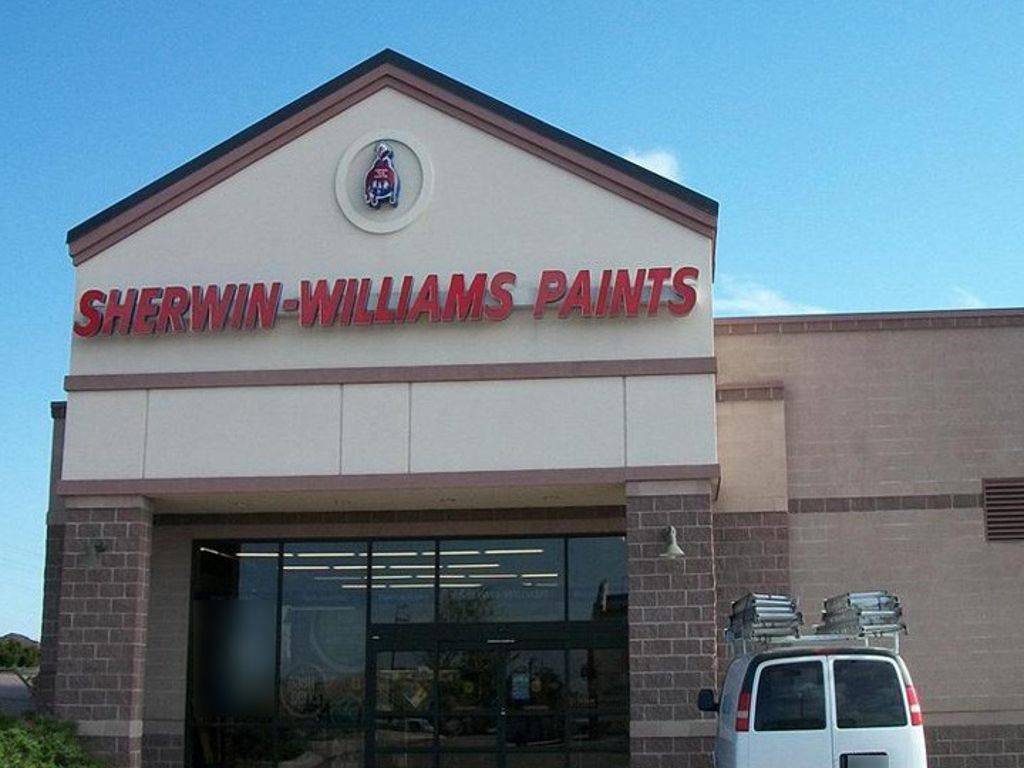The photograph captures an exterior view of a Sherwin-Williams paint store. Prominently featured is a 3D Sherwin-Williams logo, which extends outward from the front of the building, depicting the iconic image of red paint being poured over the globe. The store has a distinctive architectural design with a steepled roof that runs along the front, accompanied by brick pillars supporting an overhang area. This covered space likely provides shelter from the frequent rain in the area.

The building's facade showcases a glass front which includes floor-to-ceiling windows that are taller than the entry doors, with visible fluorescent lights and various store items seen through the slightly tinted glass. The exterior walls are painted in basic brown and beige tones, accented by dark gray roof trim with a lighter brown underside. External building lights are mounted on the upper sections of the brick pillars, enhancing the store's appearance and visibility.

A white van, equipped with a white rack holding two stacks of ladders on either side, is parked to the right of the store's right pillar. The van has black tinted windows in the rear and is positioned facing the front of the store.